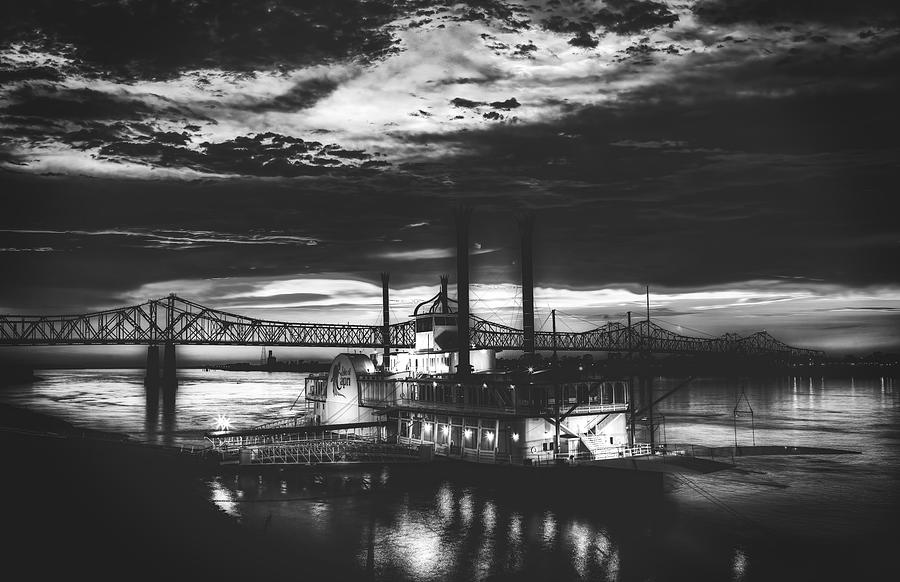This captivating black-and-white photograph captures a serene outdoor scene at dusk. Dominating the background is a grand bridge, its impressive structure spanning a vast body of water. Below, a riverboat rests, either moored at a dock or afloat, connected to the shore by intricate, silver trellis-like apparatuses. The sky, with its various shades of gray, suggests that the photograph was taken during the evening, adding a somber and tranquil ambiance. Subtle lighting illuminates parts of the background, possibly reflecting off the moon, while the riverboat itself is adorned with a few glowing lights on its lower deck, further enhancing the atmospheric mood of the scene.